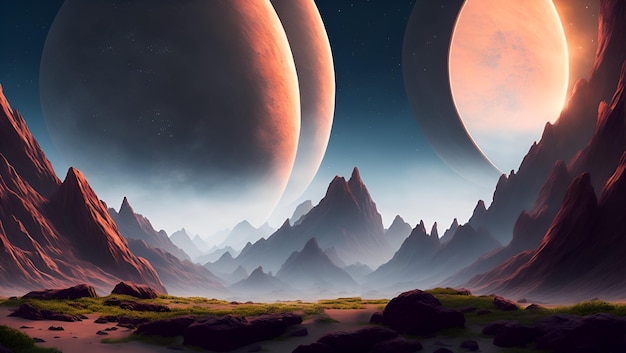The image, a piece of AI-generated digital artwork, encapsulates a science fiction landscape dominated by rugged terrain. Central to the scene is a rocky crater interspersed with sandy patches and sporadic green grass. Encircling the crater, there are tall, jagged mountains, notably one on the right that ascends to the upper edge of the artwork. The sky above features a striking arrangement of celestial bodies: two large, egg-shaped planets on the left, positioned one behind the other, and another luminescent planet to the right, half in shadow and half brilliantly lit. The backdrop gives an impression of multiple moons or planets, with at least one appearing semi-transparent and white. These elements combine to create an otherworldly, science fiction ambiance, illuminated by the stark contrast between the bright and shadowed surfaces of the celestial objects.